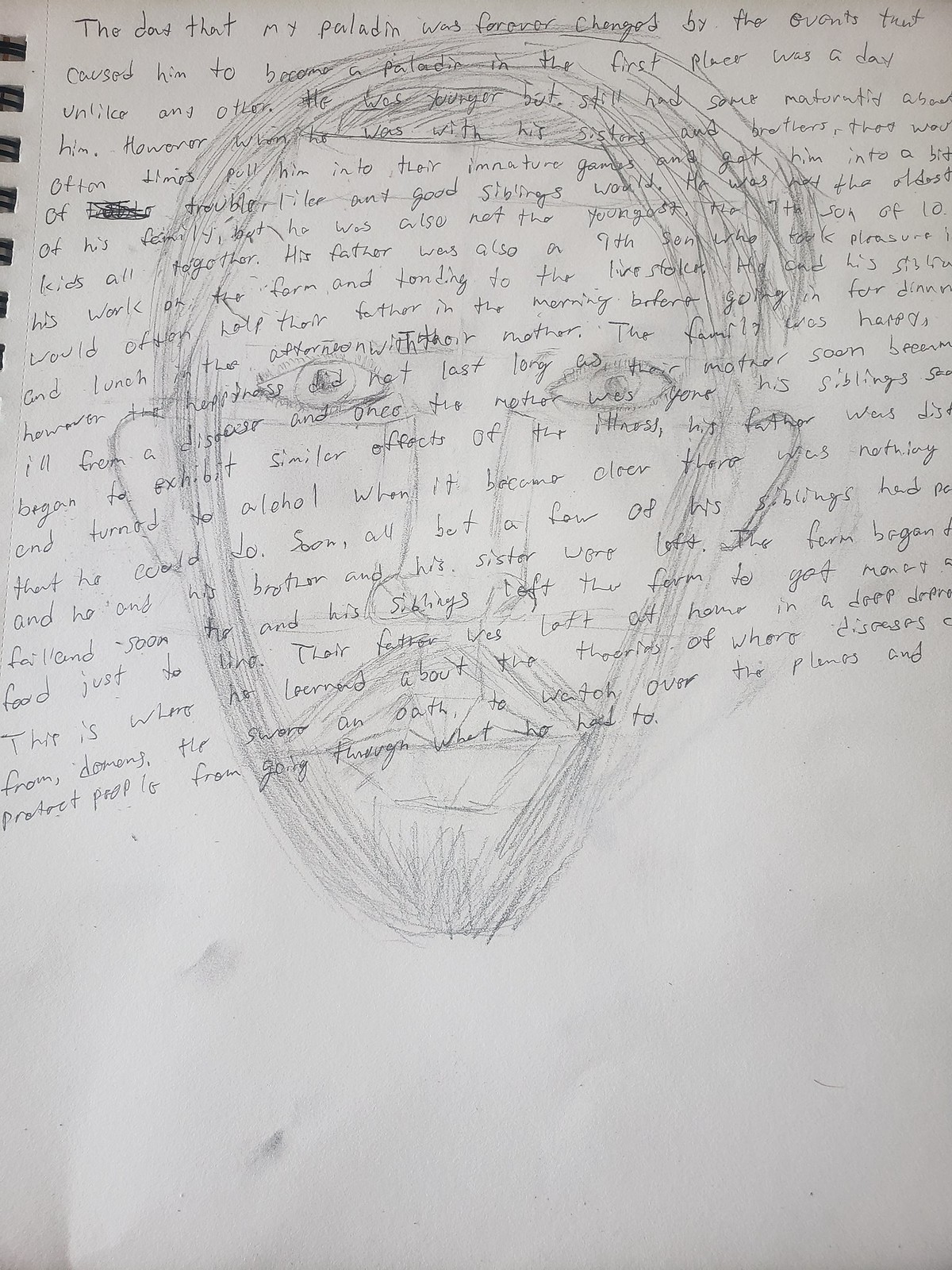The photograph captures a detailed scene of a personal journal entry written on perforated, unlined white notebook paper, hinting at deeply emotional content, possibly about someone dealing with the loss of their mother and struggling with alcohol abuse, focusing on family issues. The text is handwritten in a rather child-like scrawl, spreading across approximately 30 rows and tilting downward toward the bottom of the page due to the uneven writing. Overlapping the text is a meticulous pencil sketch of a man’s face, characterized by short hair, a short beard, and a mustache created by intricate pencil strokes. His facial features, including his large, wide nose, thick lips, small ears resembling the shape of C's, and clear, forward-looking eyes, are prominently detailed. The narrative, which appears to recount a dramatic story involving a paladin and transformative life events, is difficult to fully decipher due to the handwriting.